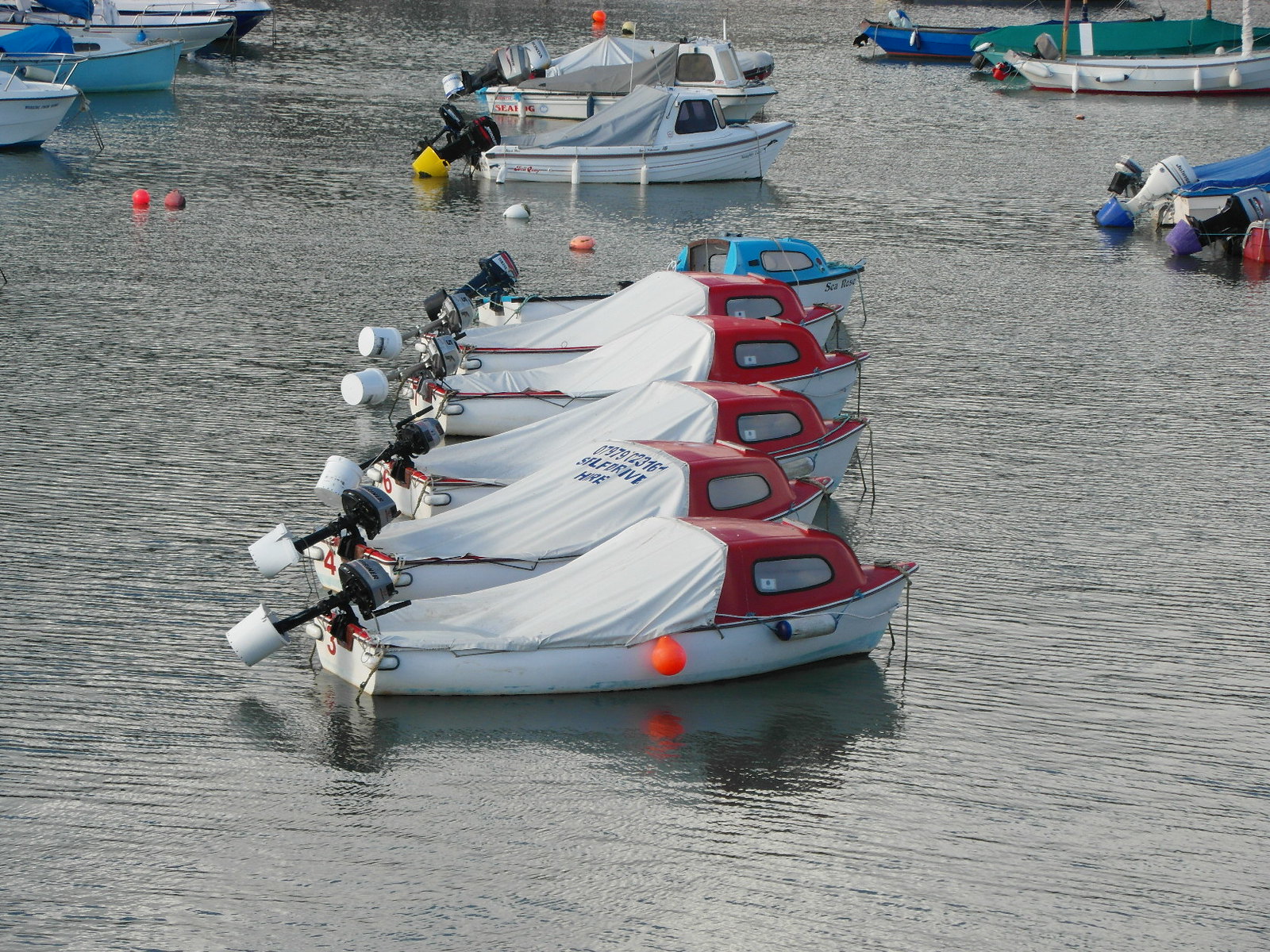This is a photograph taken from above, depicting a serene lake scene with shallow, calm water, characterized by small ripples rather than oceanic waves. About half a dozen brightly colored orange buoys float across the water. In the upper corners of the image, there are sailboats, while a distinct line of power boats stretches from the upper middle to the lower middle area. This lineup consists of five identical white boats with red cabins and lifted motors covered with protective pails, except for one boat with a turquoise blue cabin that has its motor exposed. The overall silvery reflection on the water enhances the tranquility of the scene, highlighting the boats' uniformity and the vibrant colors of their cabins. The boats not docked but parked next to each other, are flanked by other varied vessels, adding diversity to the setting with their differently colored motors and bases.